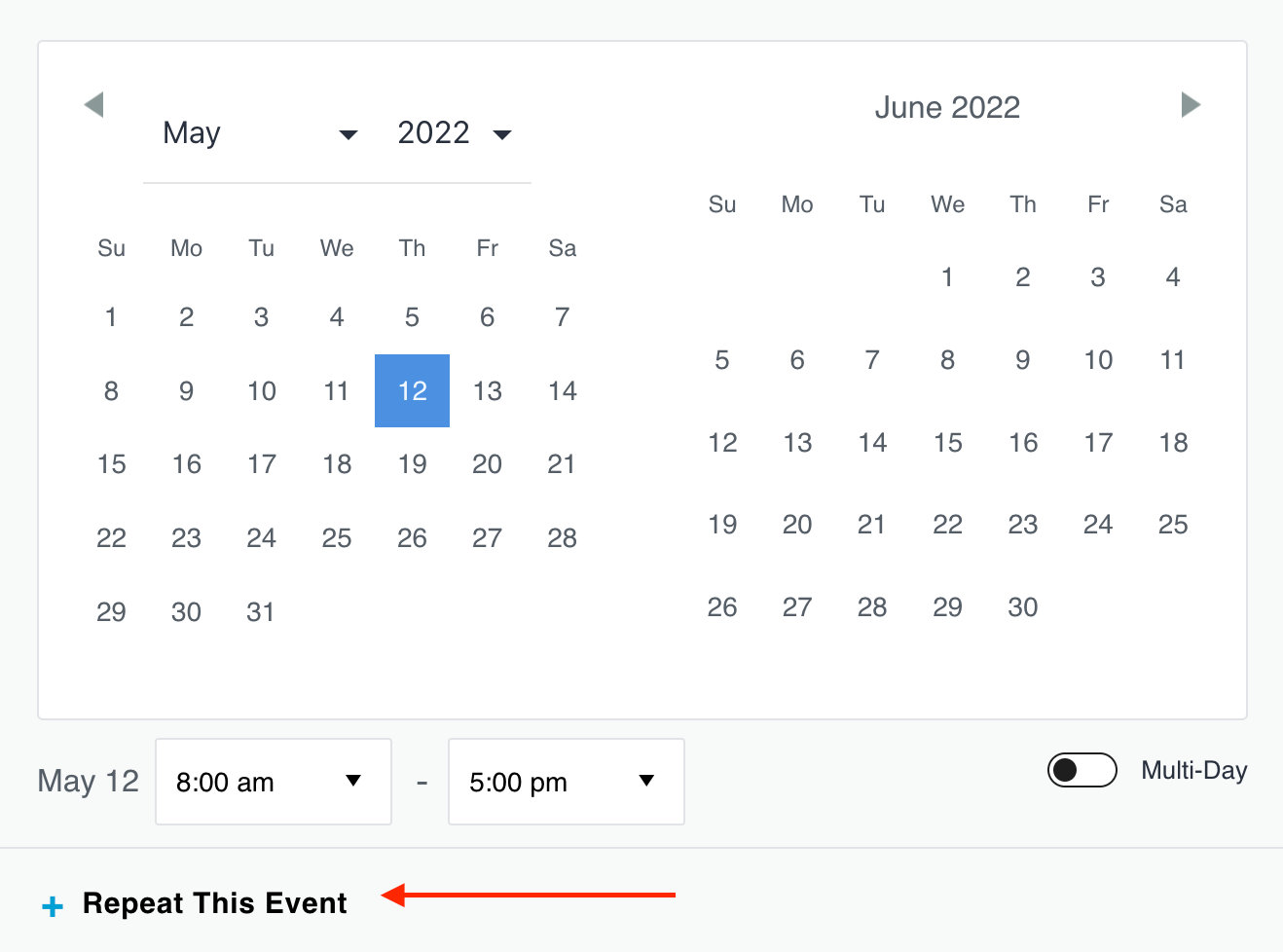Here is a detailed caption for the image:

"The image showcases a calendar interface within an app. The main section of the calendar displays two months: May 2022 on the left and June 2022 on the right. The background of the calendar itself is white, while the overall background is light gray. The month of May 2022 is presented with dates displayed from Sunday, May 1st to Tuesday, May 31st. Notably, Thursday, May 12th is highlighted, indicating a selected date. Adjacent to May, the June 2022 calendar spans from Wednesday, June 1st to Thursday, June 30th.

At the bottom of the interface, there are two drop-down boxes specifying the selected date as May 12th, with designated start and end times from 8 a.m. to 5 p.m. Additionally, a slider option is available to select 'multi-day' events. Further down, there is a plus symbol accompanied by the text 'Repeat this event,' suggesting an option to set recurring events. This image depicts an app's event scheduling feature in detail."